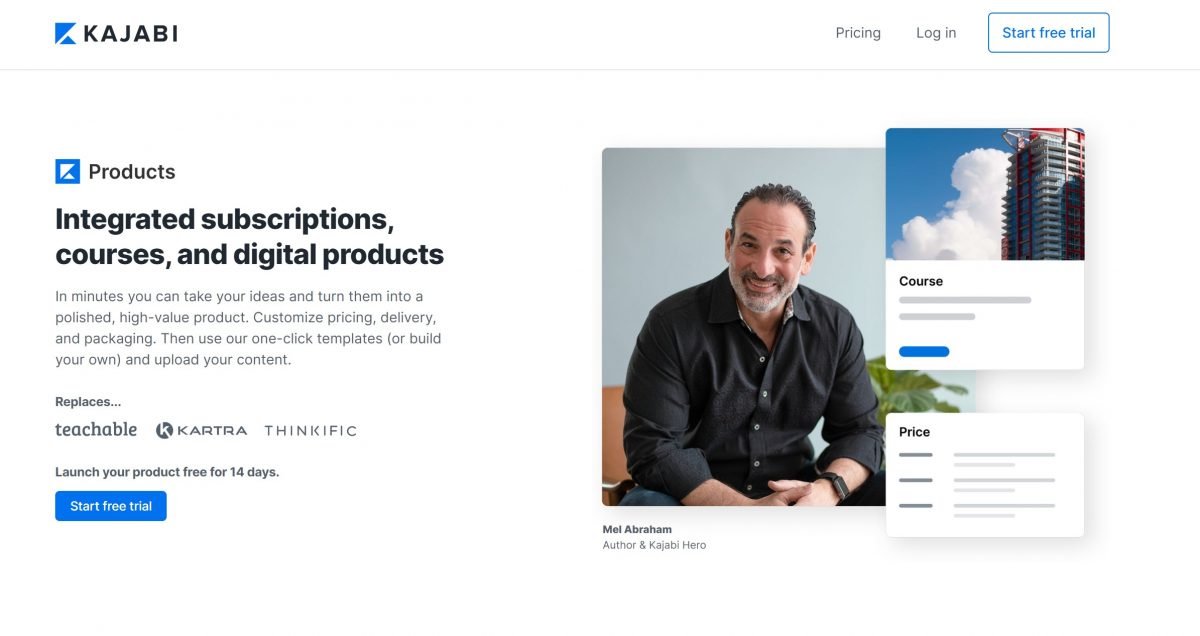The image showcases "WAPI," a platform designed for creating and managing products, integrated subscriptions, courses, and digital offerings. The main message highlights how users can quickly transform their ideas into polished, high-value products with cost-effective pricing, delivery, and packaging solutions. It emphasizes one-click templates that allow users to build their own designs and upload content, effectively replacing services like Teachable, Kartra, and Thinkific. A call to action invites users to launch their product with a free 14-day trial, personally recommended by "Blue."

On the right side of the image, there are buttons for pricing, logging in, and starting the trial. Featured prominently is Mel Abraham, an author and Kodabi hero. He is depicted as a smiling man with short, curly hair, wrinkles on his forehead, and a gray beard. He is wearing a black shirt, a black watch, and blue jeans, while clasping his hands together. The background includes a gray wall, a chair on the left, and green leaves on the right.

Additionally, the top right corner displays elements like a gray bar, a blue rectangle, a circle, an oval, and a blue sky with white clouds. Also visible is a very tall building. The bottom section of the image features pricing details on a white background with shadows in the back.